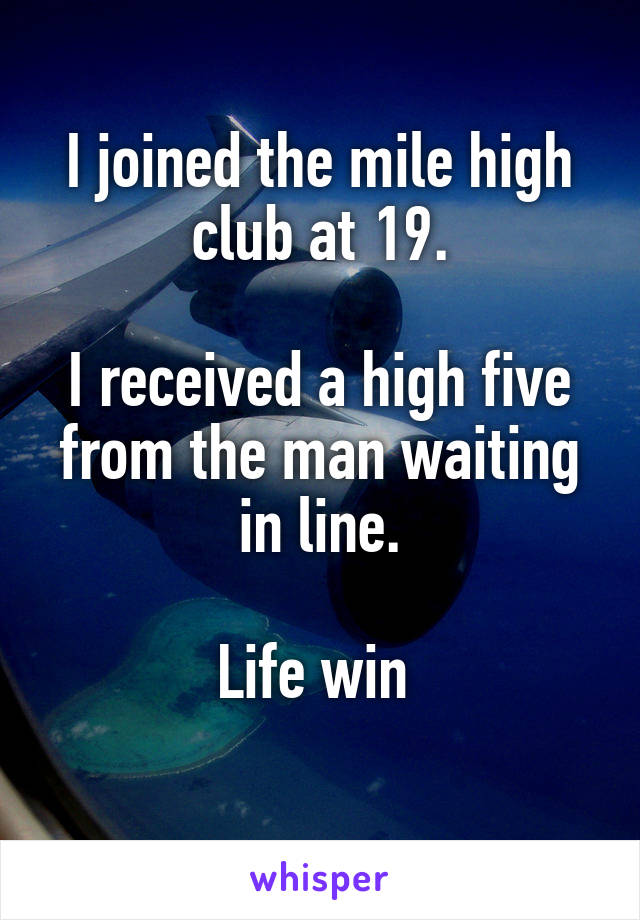The image is a vertically aligned rectangular meme featuring part of a large jet aircraft's wing with two jet engines, flying against a dynamic blue background gradient that transitions from dark blue at the top to a lighter blue in the middle, and slightly darker at the bottom. White text is prominently centered on the background, reading, "I joined the Mile High Club at 19. I received a high five from the man waiting in line. Life win." Below the main image, on a white area, the word "whisper" is displayed in purple, lowercase letters, possibly indicating the source website. In the background, the sky is dark blue with patches of white clouds and small green islands are visible below, giving the impression that the aircraft is flying over a scenic landscape, potentially man-made islands resembling those in Dubai.